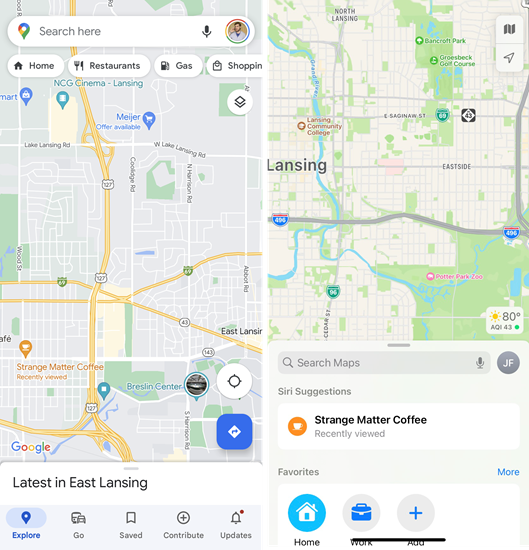The composite image showcases two screenshots from a digital map application, likely Google Maps, with detailed interface elements and map information displayed. 

The left screenshot features the top segment with a "Search here" prompt within a Google search bar. Directly beneath, there are quick-access buttons labeled "Home," "Restaurants," "Gas," and "Shopping." The main portion of the screen displays a map, complete with highways, streets, and notable points of interest such as "Meyer," "Strange Matter Coffee," and "Breslin Center." Additionally, it includes a label reading "Latest in East Lansing," indicating the area shown is East Lansing. The bottom of the screen contains navigation options: "Explore," "Go," "Save," "Contribute," and "Updates."

The right screenshot presents a map primarily focused on Lansing. This map also highlights various points of interest like "Bancroft Park," a generic label "Park," and "Grosbeck Golf Course." Below the map, a search bar reads "Search maps," with a recent search entry, "Strange Matter Coffee," indicating a previously viewed location. At the screen's bottom are buttons for "Home," "Work," and "Add," facilitating quick navigation and custom location entries.